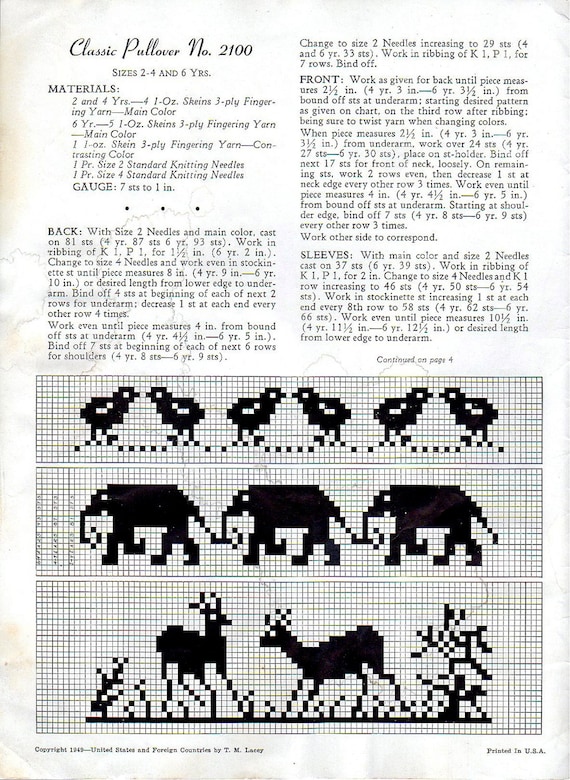This image captures a detailed page from a knitting booklet featuring the "Classic Pullover" pattern, numbered 2100, designed for children aged 2 to 4 and 6 years old. The top section includes comprehensive instructions covering materials, the back, front, and sleeves of the pullover. It specifies using skeins of yarn and size 2 needles, beginning with casting on a certain number of stitches and providing step-by-step directions for each segment. The materials list mentions a 4.1 oz skein and the pattern gauge of 7 stitches per inch.

Below the text instructions, a detailed knitting chart is presented. This chart consists of three patterned rows framed by a black and white grid, aiding in accurate stitching. The top row depicts pairs of black bird silhouettes facing each other. The middle row features black elephants, interconnected by their trunks and tails. The bottom row shows two black deer seemingly frolicking. All the animals are intricately detailed and set against a backdrop of numerous small squares, suggesting a structured approach to the design.